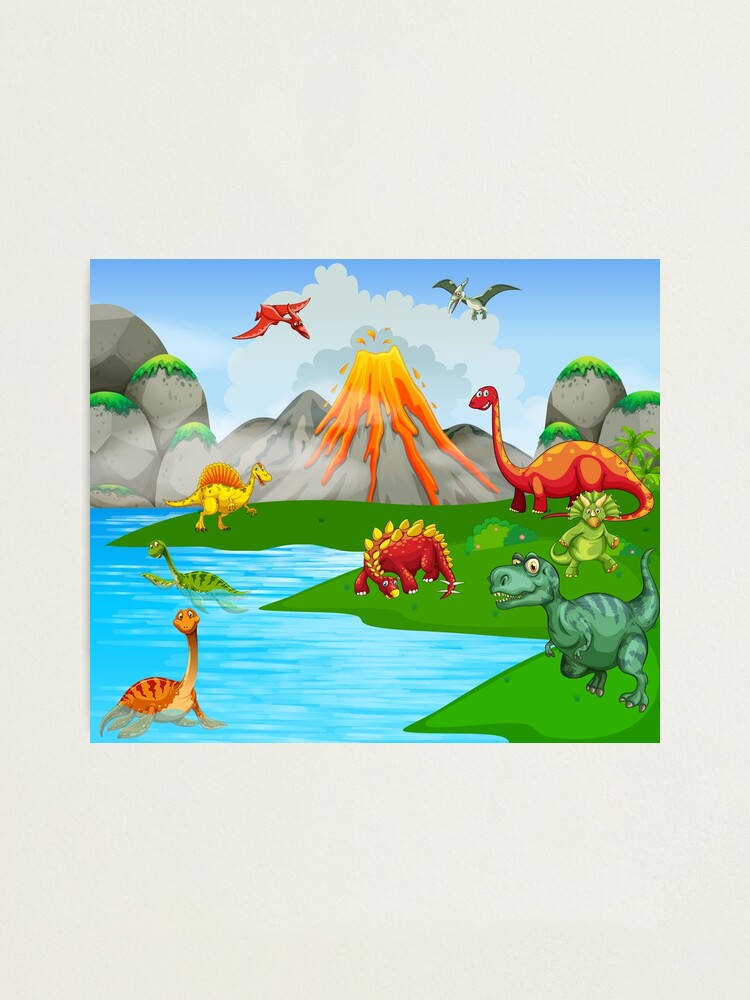In this children’s comic-style illustration, a vibrant array of dinosaurs are depicted on a lush, verdant island with a dramatic erupting volcano in the background. The volcano, located about 100 feet from the dinosaurs, spews orange and yellow lava while smoke billows into the air, yet the dinosaurs remain blissfully unaware as they cheerfully gaze at the viewer. The sky, colored in a blue gradient with occasional clouds, features pterodactyls – one red and one gray – soaring through the air. The ground is adorned with green grass and patches of rocks, creating a serene backdrop despite the volcanic activity. Surrounding the volcano, going clockwise, are various dinosaurs: an orange dinosaur, a small green dinosaur, a red dinosaur with yellow spikes (possibly an ankylosaurus), and a darker green dinosaur with green stripes. The foreground showcases a colorful cast: a green T. rex, a red brontosaurus, a green triceratops standing on its hind legs, and a yellow dinosaur with spines running down its back. Additionally, two dinosaurs swim in the adjacent blue waters, one orange and one green. All the dinosaurs, including familiar faces like Sara and Spike from "Land Before Time," are depicted with joyful expressions, seemingly waving at the observer, creating a whimsical and lively scene.